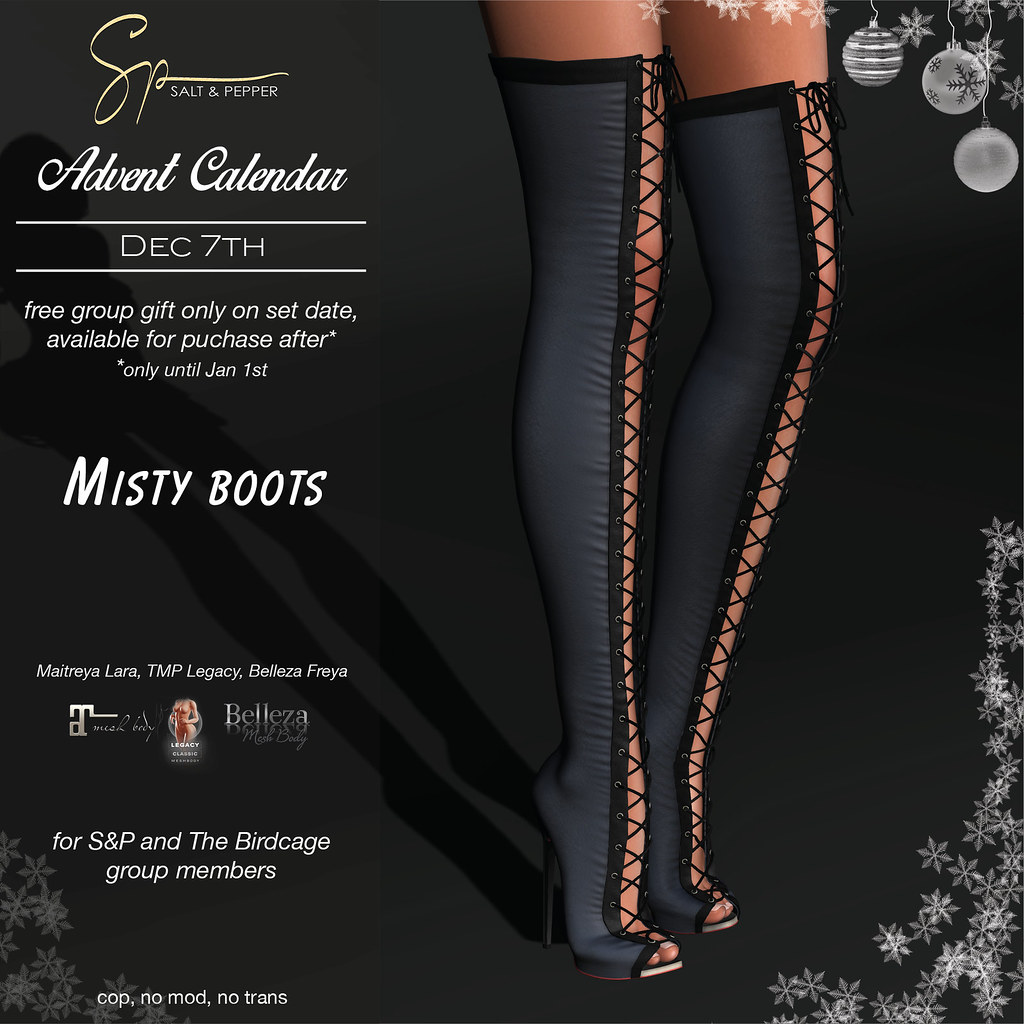The promotional material is an advertisement for a women's footwear product by the retailer "Salt & Pepper." The top left corner of the ad features a stylized "S&P" logo in light yellow, indicating the brand name. The text is somewhat hard to read but clearly says "Salt & Pepper." Below the logo, it mentions "Advent Calendar December 7th Free Group Gift," indicating a special offer available only on that date and purchasable until January 1st.

Dominating the center-right of the image is a detailed visual of the product, named "Misty Boots," showcased in large white text. The boots are depicted as high-heeled, black, thigh-high boots with an open front design, revealing the wearer's skin and held together with black laces, exuding an adult and stylish appeal. The boots appear to be intended for at-home wear rather than outdoor use. 

The background of the image is predominantly black, with festive elements adding to a holiday theme. In the top right corner, there are transparent white Christmas tree ornaments (baubles) and silver stars, while the bottom right corner features more silver stars and stacked snowflakes, emphasizing the Christmas sales event theme.

Additionally, the bottom left of the image lists compatible sizes and brands, mentioning "Maitreya, Laura, TMP, Legacy, Beleza, Freya," and indicates that the boots are available for "S&P and the Birdcage group members" with the terms "copy, no modify, no transfer."